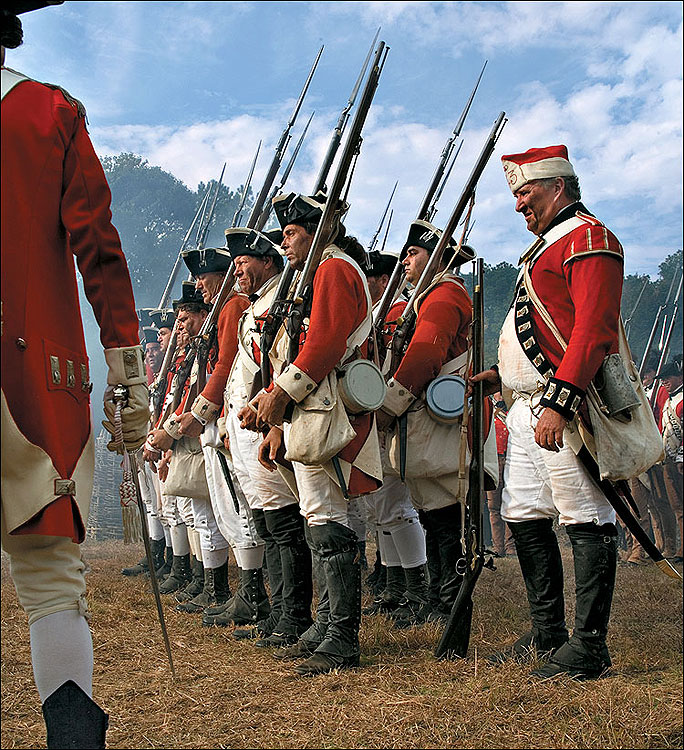The image depicts a large formation of men dressed in military uniforms, each outfit featuring a red jacket with white undershirts and white pants, complemented by either tall black boots that reach their knees or shorter ankle-high boots. The men, possibly British soldiers from the East India Company in the early 1900s, or participants in a historical reenactment, all face towards the left side of the image, standing straight and looking forward. Many soldiers are equipped with long guns, some held at their sides, while one man in the front right holds his gun on the ground. The soldiers are also adorned with a variety of hats ranging from black and white to red and white, and carry additional accessories such as cloth bags and canteens. On the far left, a commander with his back to the viewer walks forward carrying a sword. The setting is outdoors by day, with a clear blue sky, white clouds, trees in the background, and a field strewn with twigs, bushes, and grass.